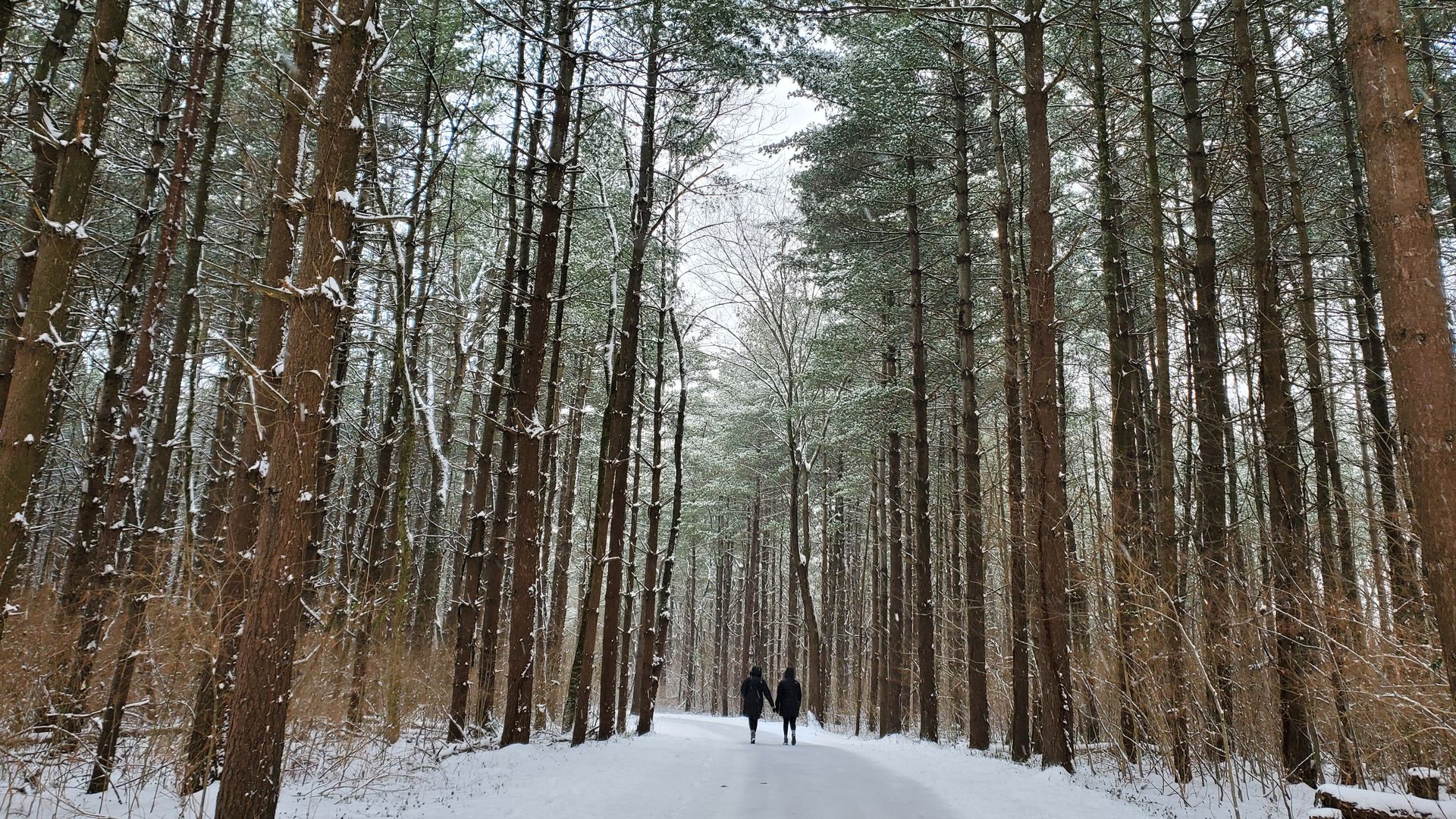This photorealistic image captures a picturesque winter scene, where a couple, dressed in black winter coats and pants, walks hand-in-hand down a snow-covered path that winds gently to the left. The path is set in the middle of a dense forest, lined with very tall, thin trees on both sides. These trees, sparse with branches until higher up, are laden with green and snow-dusted leaves, possibly pine. The ground is blanketed in snow, though the path itself appears to have a light coating, suggesting it may have been shoveled or plowed. At the bottom corners of the image, dead tree saplings with white bases and brown, dried leaves stand amidst the snow. The couple, silhouetted against the wintry landscape, are seen from behind, walking away into the distance, their figures darkening against the lightly clouded, yet bright daytime sky.